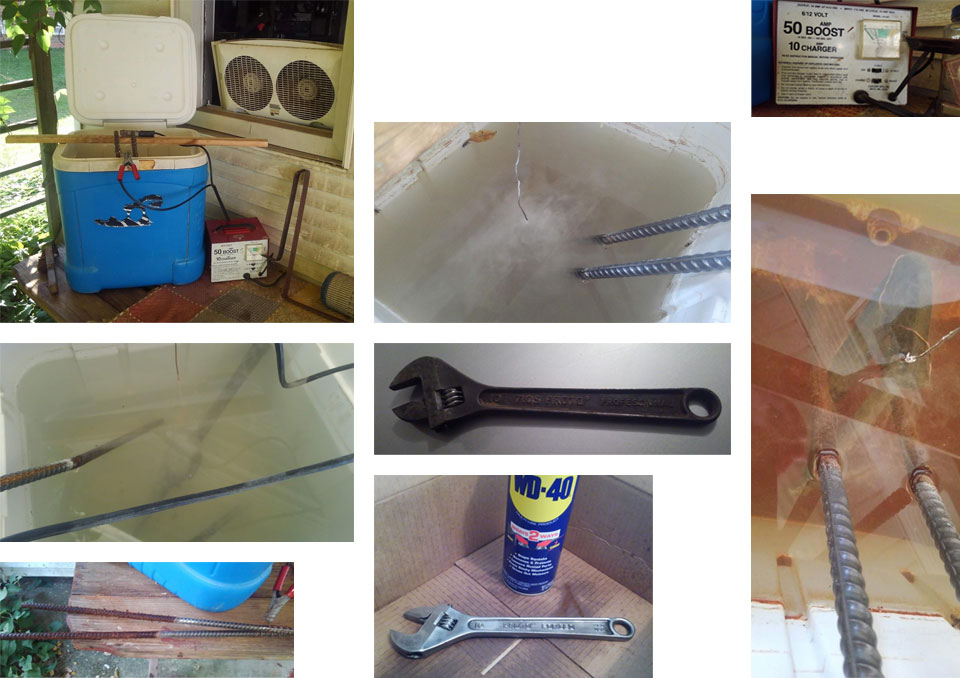The collage showcases eight different photos depicting a potentially homemade air conditioning system. The upper-left image features a blue cooler with a white lid. Across the top of the cooler, a piece of wood is positioned with two steel rods, or rebars, inserted into the cooler. A battery lies to the right of the cooler, connected by power lines. Positioned above the cooler, a window fan with two propellers faces inward.

The center-left image captures the interior of the cooler, revealing the submersed steel rods amidst some liquid. Below this, an image of a tabletop displays two steel rods or rebar pieces resting on the surface.

The middle column begins with another view of the cooler's interior, showing the submerged rods once more. Directly beneath this, an older, possibly rusty, wrench is photographed. Further down, a newer silver wrench shares the spotlight with a can of WD-40, both placed within a cardboard box against a tiled surface.

The right column starts with an image of a box labeled "50 boosts." Finally, the lower right photo depicts a semi-transparent image of a person wearing a bluish-green outfit, shown in a reflective surface alongside two vertically placed steel rods, giving an impression of depth and layering within the composition.

Each image collectively builds a comprehensive view of a homemade air conditioning system, emphasizing the utilization of everyday materials and tools in its assembly.